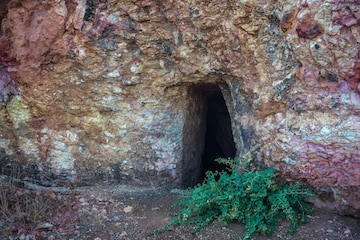This image depicts a slightly mysterious entrance to a cave or hewn-out doorway within a solid stone or mountainside, measuring approximately 4 to 5 feet in height. The entrance, which is quite narrow and keyhole-shaped, can accommodate only one person at a time. Surrounding the entrance are multi-colored rocks, displaying a remarkable array of hues including various shades of red, orange, rose, pink, white, and even a pearlescent blue. This rainbow-like coloration appears strikingly unnatural. Just in front of the opening lies a lush green plant with long, fern-like leaves on a ground scattered with red and brown rocks and dirt. The interior beyond the doorway is shrouded in darkness, giving no hint of what lies within.